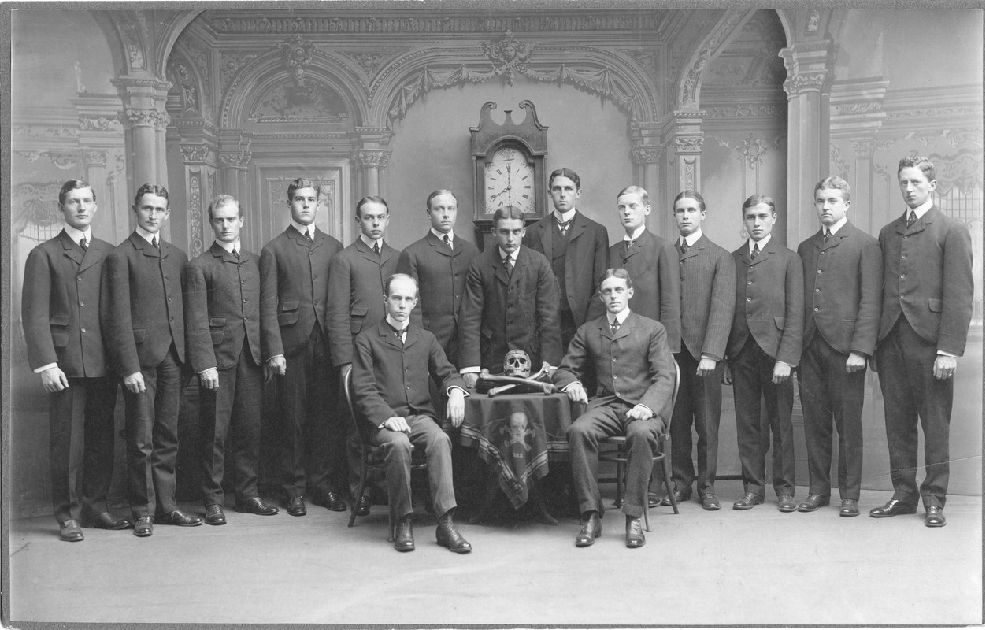This black-and-white landscape-style photograph, likely taken in the early 1900s, showcases a group of 15 men. Thirteen men stand in a straight row, all dressed in dark suits and sporting short hair, directly facing the camera with stern expressions. In front of them, two men sit on ornate chairs, their demeanor equally serious. Between the seated men, a small round table is prominently displayed, draped with a tablecloth adorned with a skull and crossbones motif. Atop the table rests an actual skull and crossbones, adding a macabre touch to the scene. Both seated men have their arms placed on the table, further emphasizing its central significance in the photograph. The composition and attire suggest a formal gathering, possibly a historical fraternity, secret society, or a commemorative assembly.